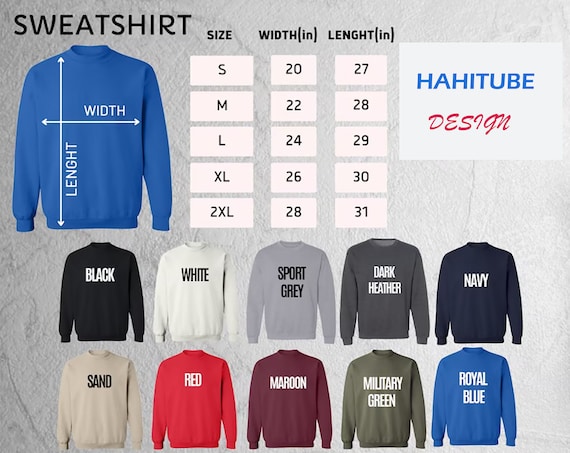This image is an advertisement layout for sweatshirts. At the top, the heading "Sweatshirt" is prominently displayed in black print. Below this, there is a detailed size chart that includes measurements for Small, Medium, Large, Extra Large, and 2XL sizes. The dimensions are listed as follows: Small (20 inches width, 27 inches length), Medium (22 inches width, 28 inches length), Large (24 inches width, 29 inches length), Extra Large (26 inches width, 30 inches length), and 2XL (28 inches width, 31 inches length). On the left side, a blue sweatshirt is illustrated with arrows indicating its width and length. Above this illustration, the text "Haha Tube Design" is displayed. The background of the image is gray, and below the size chart and sweatshirt illustration, there is a showcase of the available sweatshirt colors. These colors include black, white, sport gray, dark heather, navy, sand, red, maroon, military green, and royal blue, displayed in a row. Each color swatch is neatly aligned, providing a visual representation of the available options.